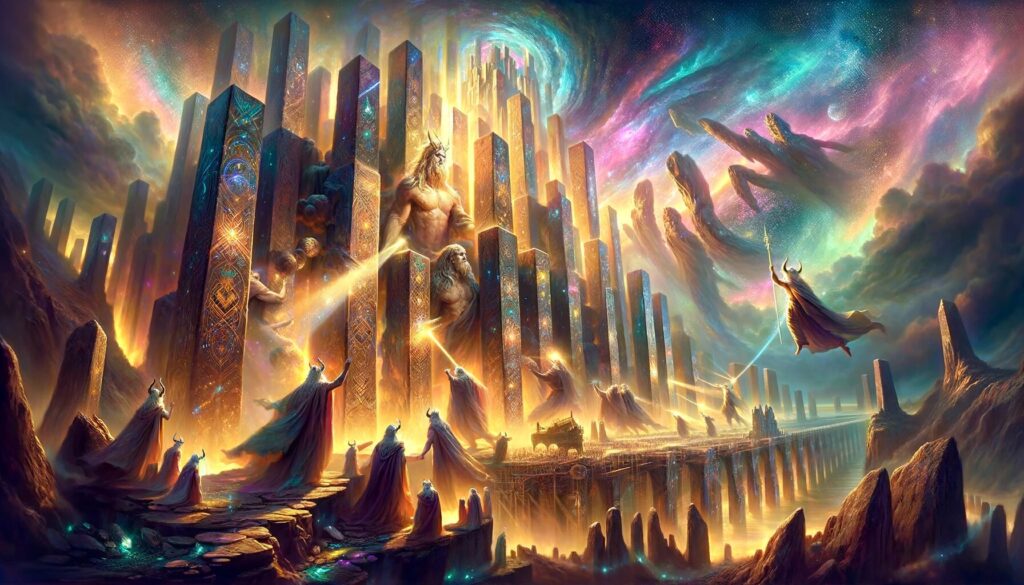In this intricately detailed illustration, a mystical scene unfolds featuring several god-like figures adorned in flowing robes. These ethereal beings have light-colored hair and some possess horns, exuding an aura of divine presence. They stand majestically on rock outcroppings, surrounded by glowing objects emitting shades of purple, teal, and gold. Towards the top of the image, luminescent columns in teal, purple, gold, and pink light the scene, enhancing its otherworldly atmosphere.

Amidst this celestial gathering, a few seated deities command attention. One, with a beard and flowing white hair, exudes wisdom, while another, sporting flowing hair and horns, radiates a powerful, enigmatic energy. These figures are embraced by the glowing columns of light and flanked by caped figures that add to the scene's grandeur.

The sky above swirls with vibrant colors—teal, pink, gold, magenta, and purple—creating an aura of both beauty and ominous intensity. Below, more rock formations rise from the ground, completing the composition of this captivating and mystical tableau.